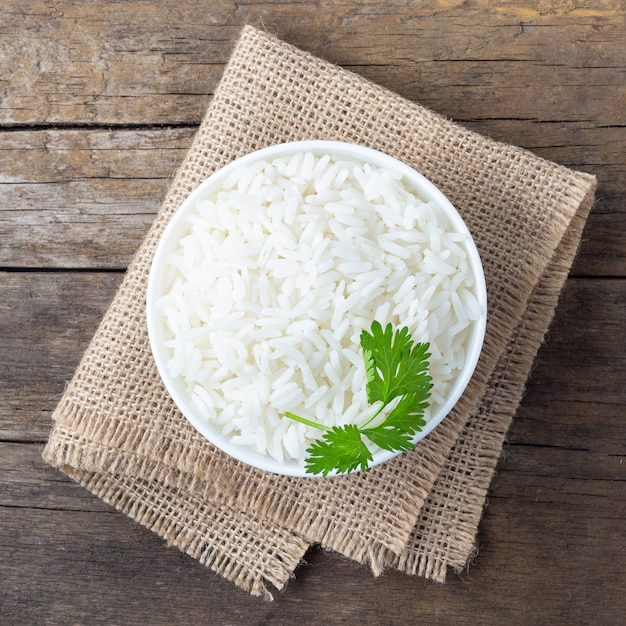This professionally shot photograph showcases a white bowl filled with long-grain white rice, placed on a rustic, woven tan tablecloth. The tablecloth features a loose weave and frayed edges, folded over twice, creating a textured backdrop. Sitting on a worn wooden table, the surface displays natural patterns and cracks, contributing to the scene's rustic aesthetic. The bowl of rice is adorned with a single green sprig, possibly cilantro or parsley, meticulously selected for an appetizing presentation. The overall composition, lighting, and texture of the items in the photograph emphasize a harmonious blend of simplicity and rustic elegance.